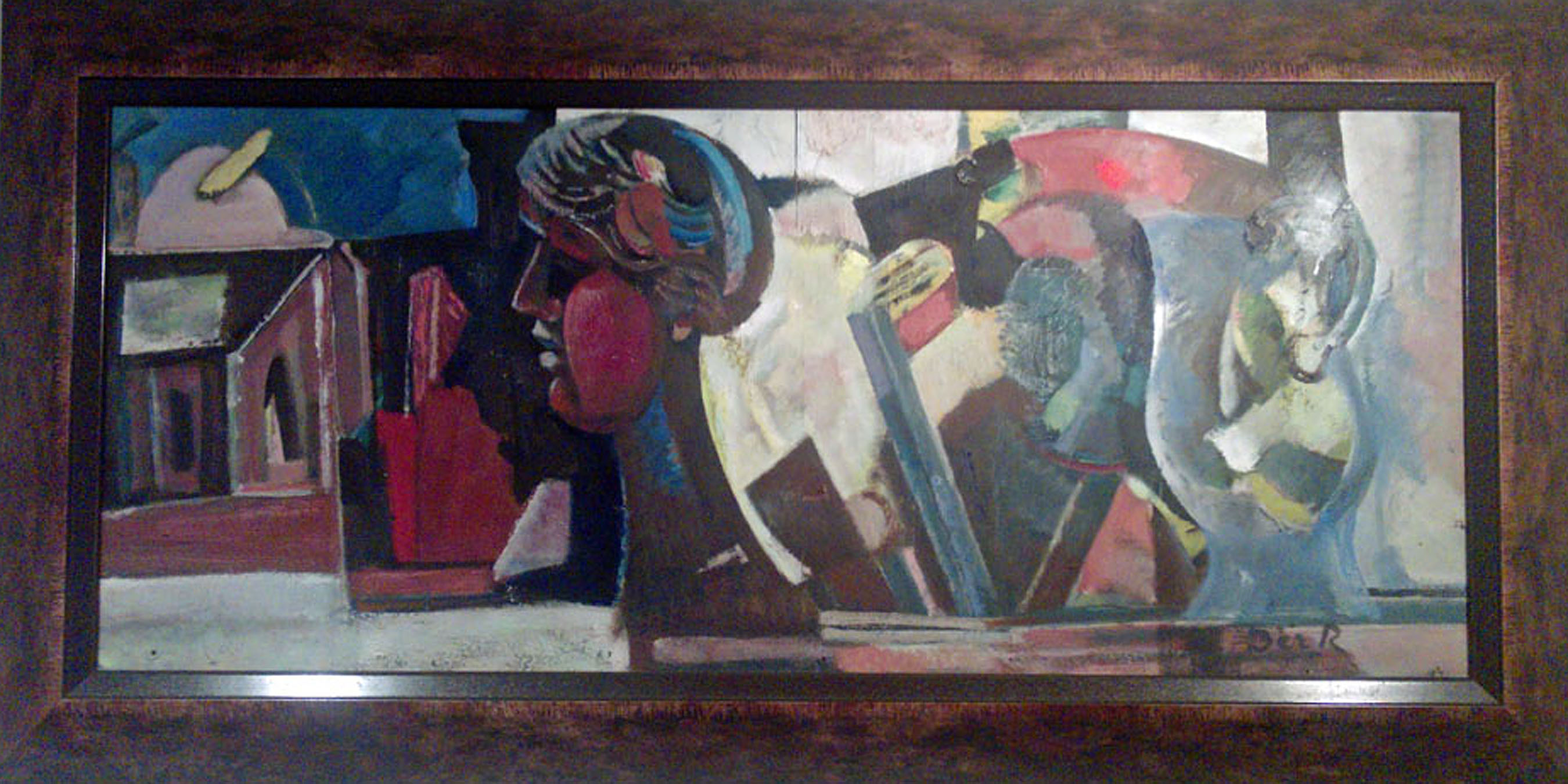This is a horizontally oriented, rectangular surreal painting encased in a dark brown wooden frame with a black inner border. The artwork is predominantly in tones of bright red, vivid blue, white, cream, black, dark green, and light green, with various abstract and surreal elements. The painting features several key elements: starting from the left, there is a blue sky with a moon and a red barn. Adjacent to it is a black silhouette of a building with a chimney. Centrally, a human face in side profile with swelled red cheeks and an abstract headdress dominates the scene. Within the head’s shape, there is a smaller figure of a seated woman. Surrounding this central figure are abstract shapes, swirls, and designs in multiple colors. Toward the right, a glass pitcher-like object contains another woman in a yellow dress. The painting also features a brown house with a skylight and includes red, blue, and diagonal blue rectangle shapes. At the bottom of the painting, there is writing that appears to read "DUR".